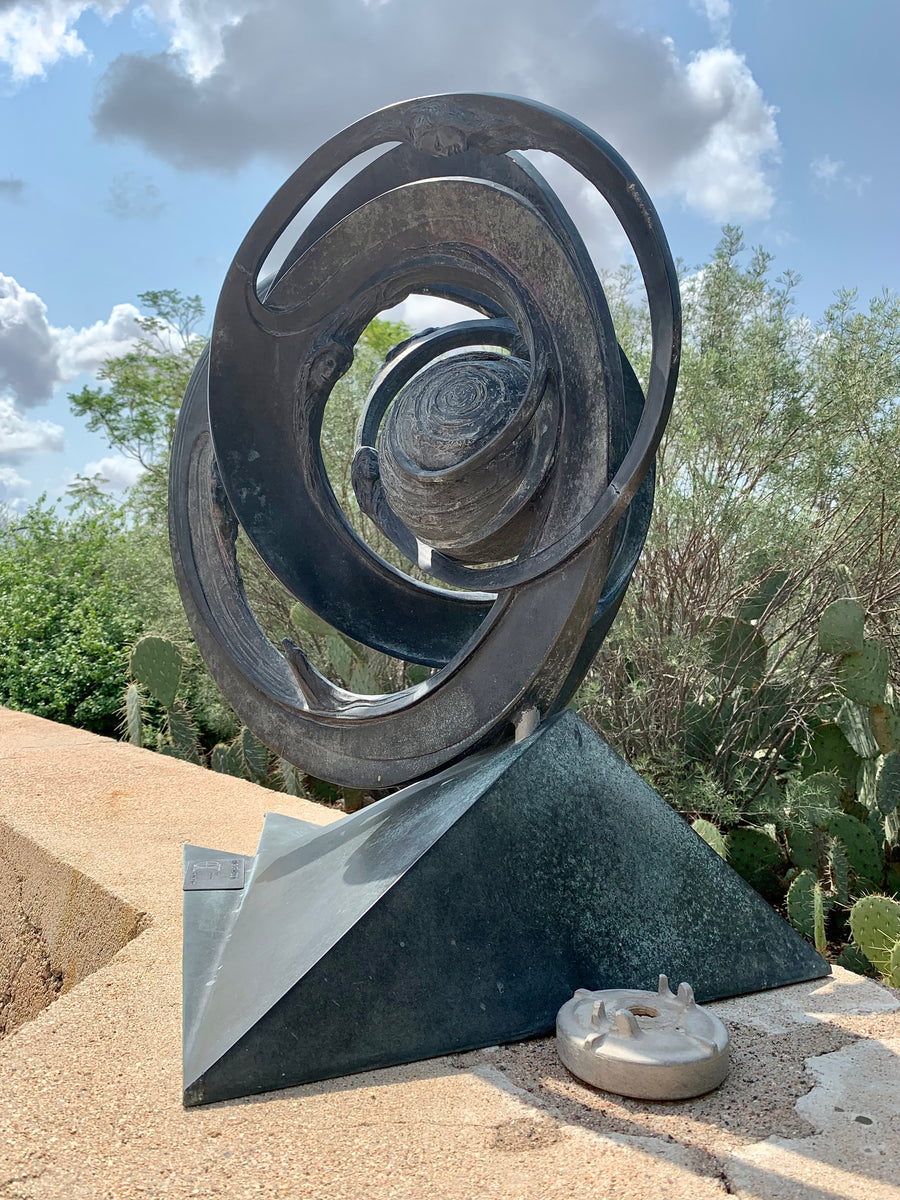This photograph captures a peculiar metal sculpture situated outdoors, prominently mounted atop a tan-colored concrete wall that extends horizontally in a long rectangle. The sculpture itself is composed of dark gray metal, showcasing a pyramid-like base that notably leans slightly to the right. Atop this base, the structure evolves into multiple intricate circles and rings, arranged in a layered and somewhat haphazard fashion. The central feature of the sculpture is a tight cluster of these concentric circles. Surrounding the sculpture, the background reveals diverse vegetation, including shrubs, trees, and distinctive cacti with oval leaves covered in thorns, suggesting a garden setting. The sky overhead is partly cloudy, featuring a mix of gray and white clouds against patches of blue. Adjacent to the sculpture, on the same concrete slab, there's a peculiar cream-colored cylindrical object adding to the scene's enigmatic ambiance.